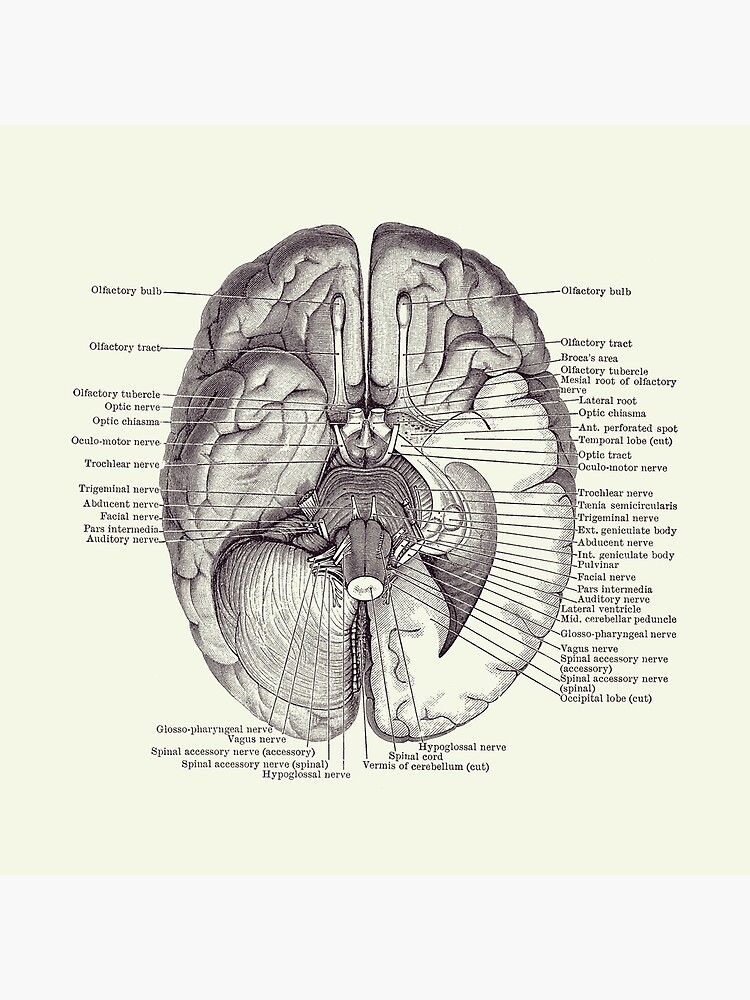The image is a detailed, vintage-style educational diagram of the human brain and nervous system, set against a soft gradient background that transitions from pale greenish-yellow to gray. It showcases a view of the brain as if seen from below, with an extensive array of labels—around 40 to 50 in total—identifying various anatomical structures. Notable labels include the olfactory bulb, olfactory tract, olfactory tubercle, lateral root, facial nerve, spinal cord, vagus nerve, Broca's area, temporal lobe, optic tract, trigeminal nerve, pulvinar, and auditory nerve. The labels are meticulously placed, covering different sections of the brain and nerves, primarily along the left, right, and bottom edges of the diagram. The detailed rendering and comprehensive labeling suggest that this image is likely sourced from an academic textbook.